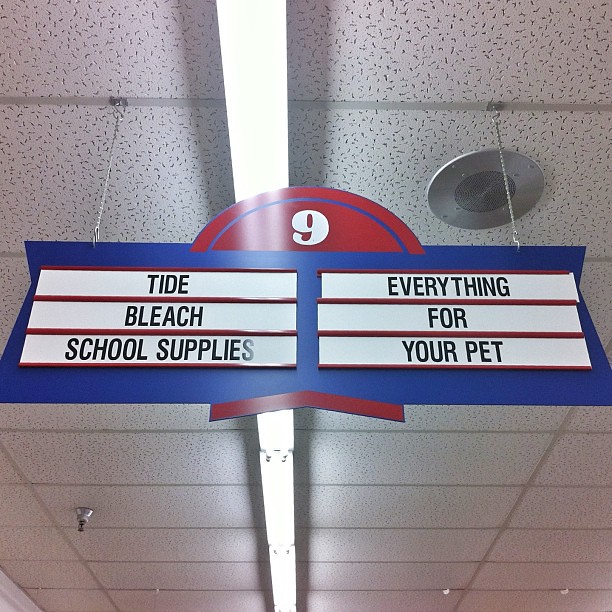An aisle in a large retail store, possibly a Walmart or a department store, featuring light gray ceiling boards with small perforations, long fluorescent lights running down the center, and round silver air vents. In the background, a large circular red sign with a blue stripe at the top prominently displays the white number "9." Another sign, blue with white stripes bordered in red and black lettering, lists product categories with "Tide, Bleach, and School Supplies" on one side and "Everything for Your Pet" on the other.